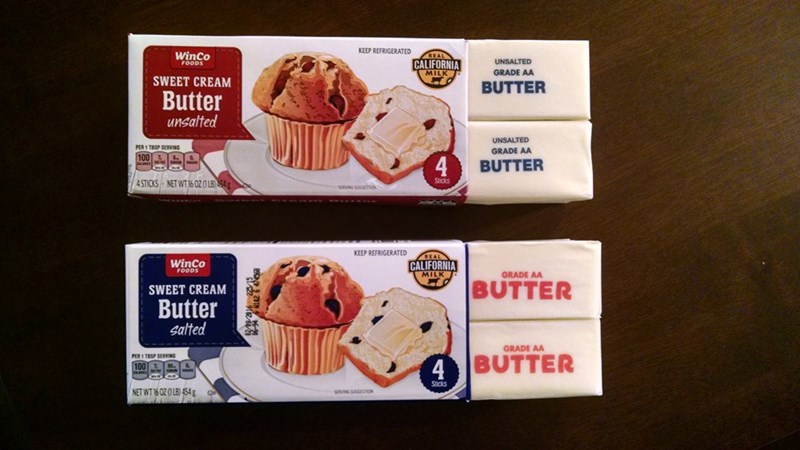The image showcases two opened boxes of Winco Foods Sweet Cream Butter—one unsalted and the other salted—arranged on a brown wooden table. Each box prominently features the red Winco Foods logo and the labeling “Sweet Cream Butter” is colored to match the type: red for unsalted and blue for salted. Both boxes display a clear image of a muffin beside a sliced piece of muffin with a pat of butter melting on it. The top box, unsalted, reveals a plain muffin on a white plate with a red-and-white cloth beneath it. In contrast, the salted butter box showcases a blueberry muffin. The boxes indicate that each contains four sticks of butter and highlight their nutritional value of 100 calories per tablespoon. Additional markings on both packages include “Keep Refrigerated,” the Real California Milk seal depicting a cow, and the “Grade AA Butter” certification.